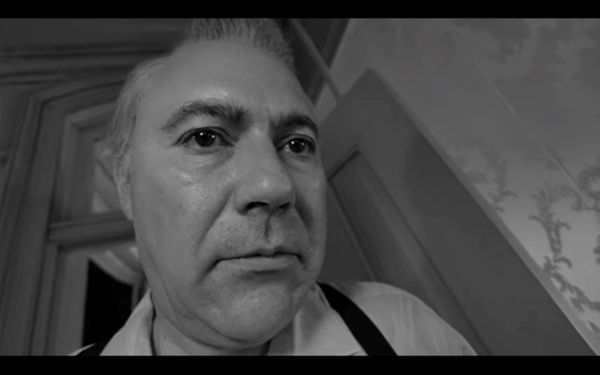This black and white photo is a close-up of a middle-aged white man, showing his face from slightly below, which includes part of his shoulders and up to his chin. He appears to be between 50 and 55 years old with dark, bushy eyebrows, wispy gray hair, and dark eyes. He's clean-shaven and looks quite sad or distressed, gazing into the distance rather than directly at the camera. The man is dressed in a white shirt with black suspenders. The backdrop suggests an older house from the turn of the 19th century, characterized by ornate wallpaper with a leafy design, heavy wooden shutters, crown molding, and wood-framed arches around the windows. There is an open door behind him, likely leading outside, as indicated by the darkness that suggests it might be nighttime. The photograph captures a sense of historical melancholy, emphasized by the man's somber expression and the intricate, old-fashioned décor surrounding him.